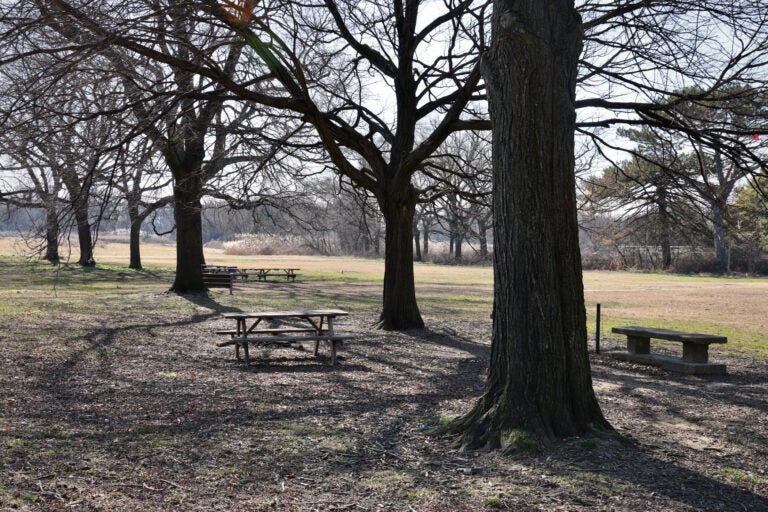This photograph depicts a serene park setting predominantly featuring thick, leafless trees, suggesting a winter scene. Dominating the foreground on the right side is a large tree trunk that extends from the bottom to the top of the image, partially obscuring its limbs and branches. The ground below exhibits a mixture of brown sand or dirt and scattered patches of dry, yellowish grass, hinting at the season. Nestled around the base of the central tree and throughout the image are several benches, some of which are linked to picnic tables. The benches vary in material, with some made of stone and concrete. To the left and middle of the image, additional trees stretch their limbs visibly, surrounded by more picnic tables. A vast field extends into the background, bordered by more thick trees, and the blue sky peeks through the foliage, providing a tranquil backdrop. In the distance, some long weeds suggest further grassland or natural park terrain.